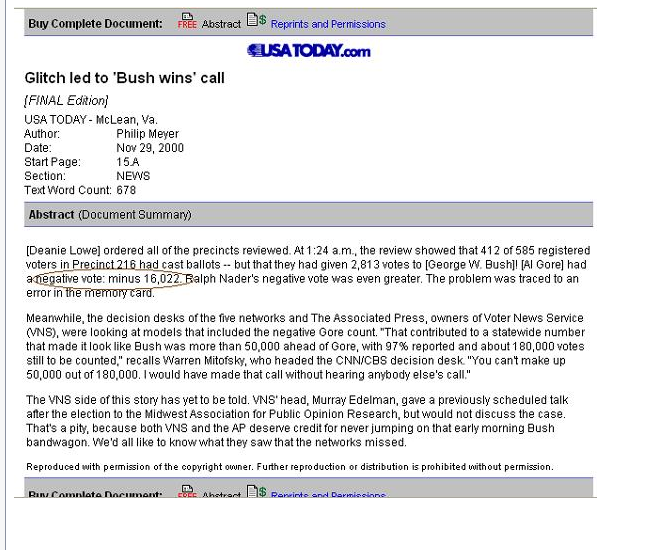The image is a detailed screenshot of an article from USA Today, specifically from the website USAtoday.com. The header features a gray bar with options like "buy complete document," "free abstract," and "reprints and permissions." The title of the article is in black text: "Glitch Led to Bush Win's Call." Below the title, in italics, it states "final edition," followed by the publication details: "USA Today, McLean, Virginia. Author: Philip Meyer. Date: November 29, 2000. Start page: 15A. Section: News. Total text word count: 678." The article's abstract summarizes that at 1:24 a.m., Deanne Lowe ordered all precincts to be reviewed, revealing significant anomalies. Precinct 216's 412 registered voters cast 813 votes for George W. Bush and a negative 16022 votes for Al Gore, alongside an even greater negative vote for Ralph Nader, due to an error traced to a memory card malfunction. At the bottom of the abstract, it notes: "Reproduced with permission of the copyright owner. Further reproduction or redistribution is prohibited without permission." The text continues below, indicating that it is part of a detailed reprint.